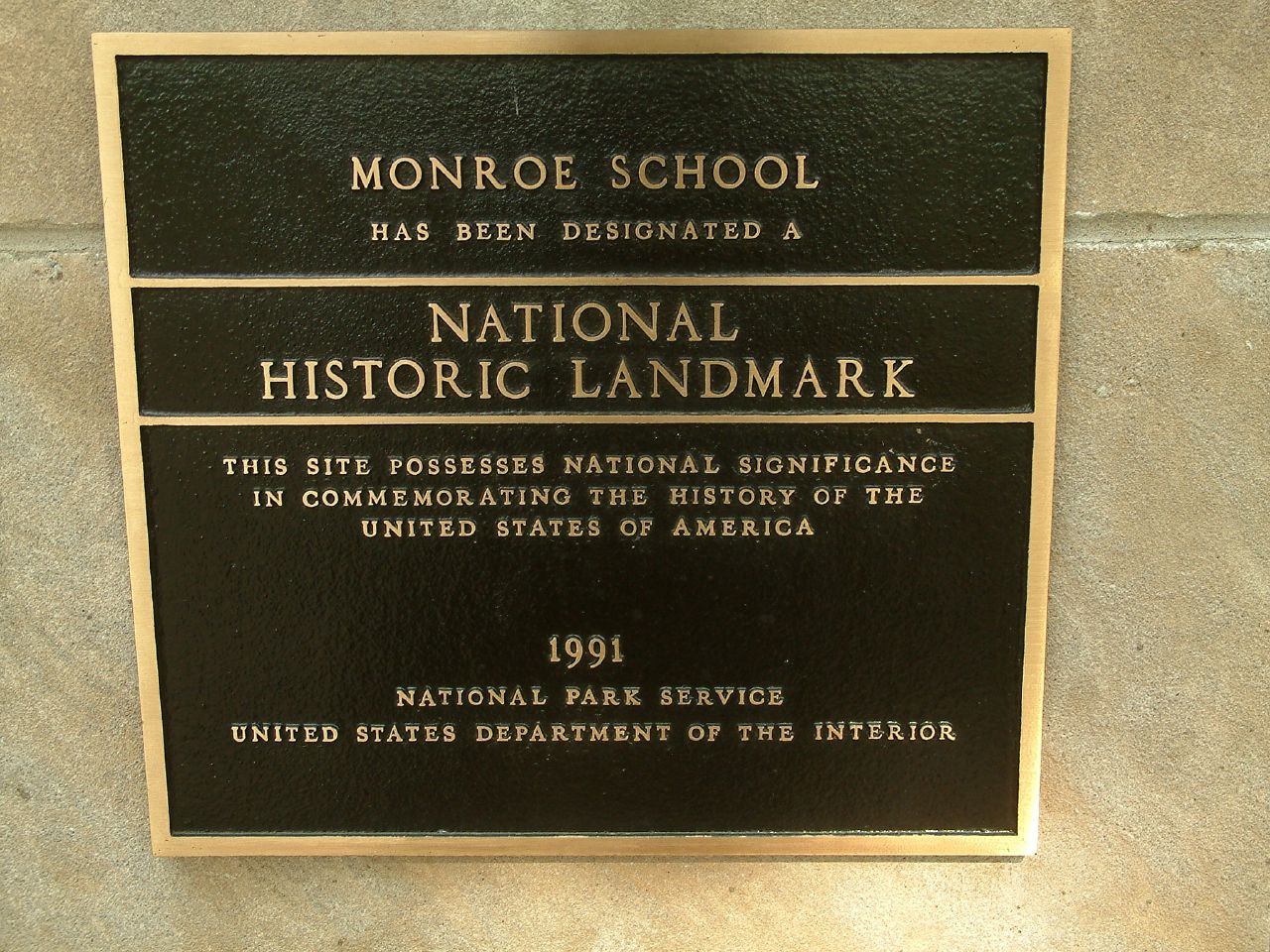In this photograph, a plaque hangs prominently on a historic stone building that has a distinct yellow hue. The plaque itself features a rich golden border and a background of brown or black, blending harmoniously with the building's color palette. The central text, all in uppercase and glistening in gold, reads: "MONROE SCHOOL HAS BEEN DESIGNATED A NATIONAL HISTORIC LANDMARK. THIS SITE POSSESSES NATIONAL SIGNIFICANCE IN COMMEMORATING THE HISTORY OF THE UNITED STATES OF AMERICA." Below this, the plaque indicates its establishment in 1991 by the "National Park Service, United States Department of the Interior." The detailed golden lettering against the dark background, framed by an ornate gold border, makes the plaque both informative and visually striking, underscoring the importance of Monroe School in the nation's history.